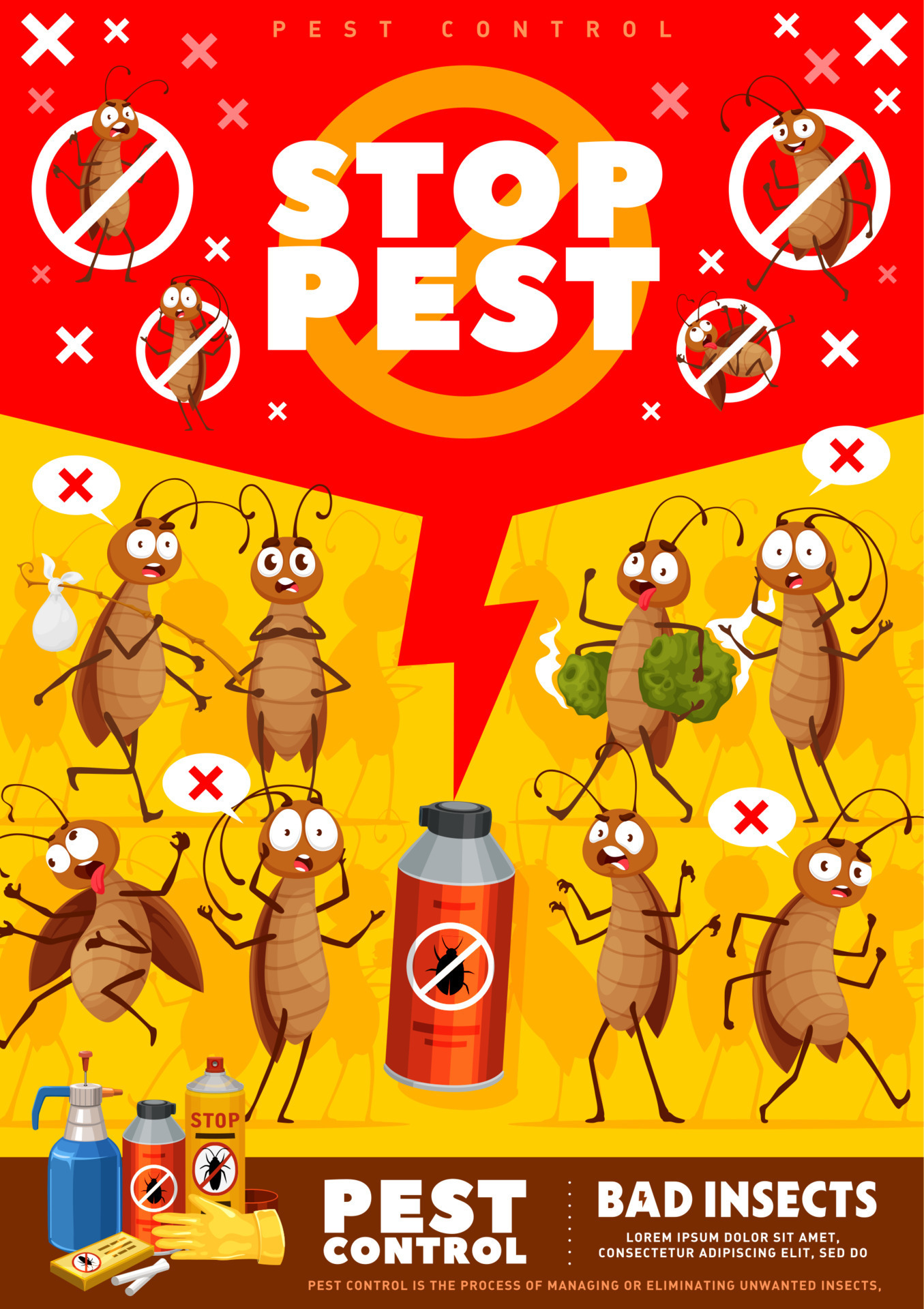"An eye-catching advertisement for pest control is dominated by vibrant red and orange hues at the top. The upper section of the poster features a prominent symbol—a white circle with a line through it—accompanied by the words 'STOP PEST' in bold, white capital letters. Below this, an arrow directs attention toward a central red can of bug spray that bears the same symbol of a bug crossed out. Surrounding the can, various cartoon bugs are depicted with X's over them, highlighting their elimination. This indicates that the spray is highly effective at killing all kinds of pesky insects. Further down, a brown banner reads 'Pest Control Bad Insects' followed by placeholder text. The poster details that pest control is essential for managing or eradicating unwanted insects, which can cause significant problems around the home. It also visually suggests that this can of pest spray can eliminate pests efficiently, making it an indispensable tool for maintaining a pest-free environment."